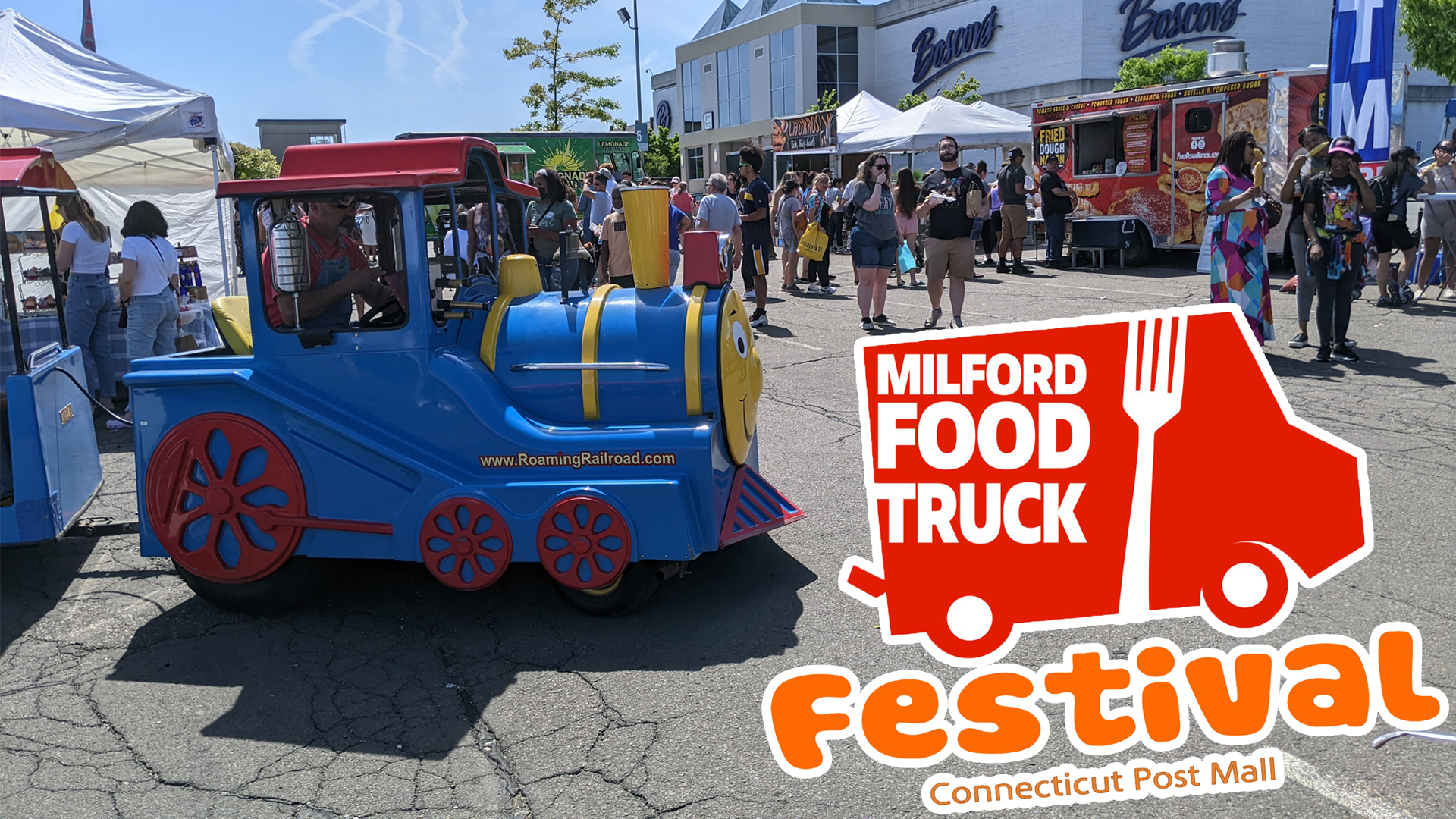The photograph used for the advertisement captures a vibrant outdoor scene on a sunny day with a partly cloudy sky. At the heart of the image is a graphic of a striking red food truck adorned with a stylized white fork and the words "Milford Food Truck," promoting the "Milford Food Truck Festival." Below the truck, highlighted in orange with a white outline, the text reads "Festival," and the location is identified at the bottom as "Connecticut Post Mall." The bustling background reveals a lively food truck festival taking place in the parking lot outside a recognizable Boscov's department store, suggesting the setting within the Connecticut Post Mall. The area is alive with an array of food trucks and white pop-up tents, while a diverse crowd of people, including individuals from different races, are seen standing in line, walking, holding food, and exploring the offerings.

A notable feature of the scene is a child-friendly novelty train, reminiscent of Thomas the Tank Engine, brightly painted in primary blue, yellow, and red hues, with a cheerful face on its front. The train, labeled with the URL www.roamingrailroad.com, is driven by a man in overalls and a red shirt and is intended to transport attendees around the festival. The small train includes additional carts for passengers, contributing to the festive and playful atmosphere. Overall, the image encapsulates the essence of a vibrant, family-friendly event brimming with culinary delights and community engagement.